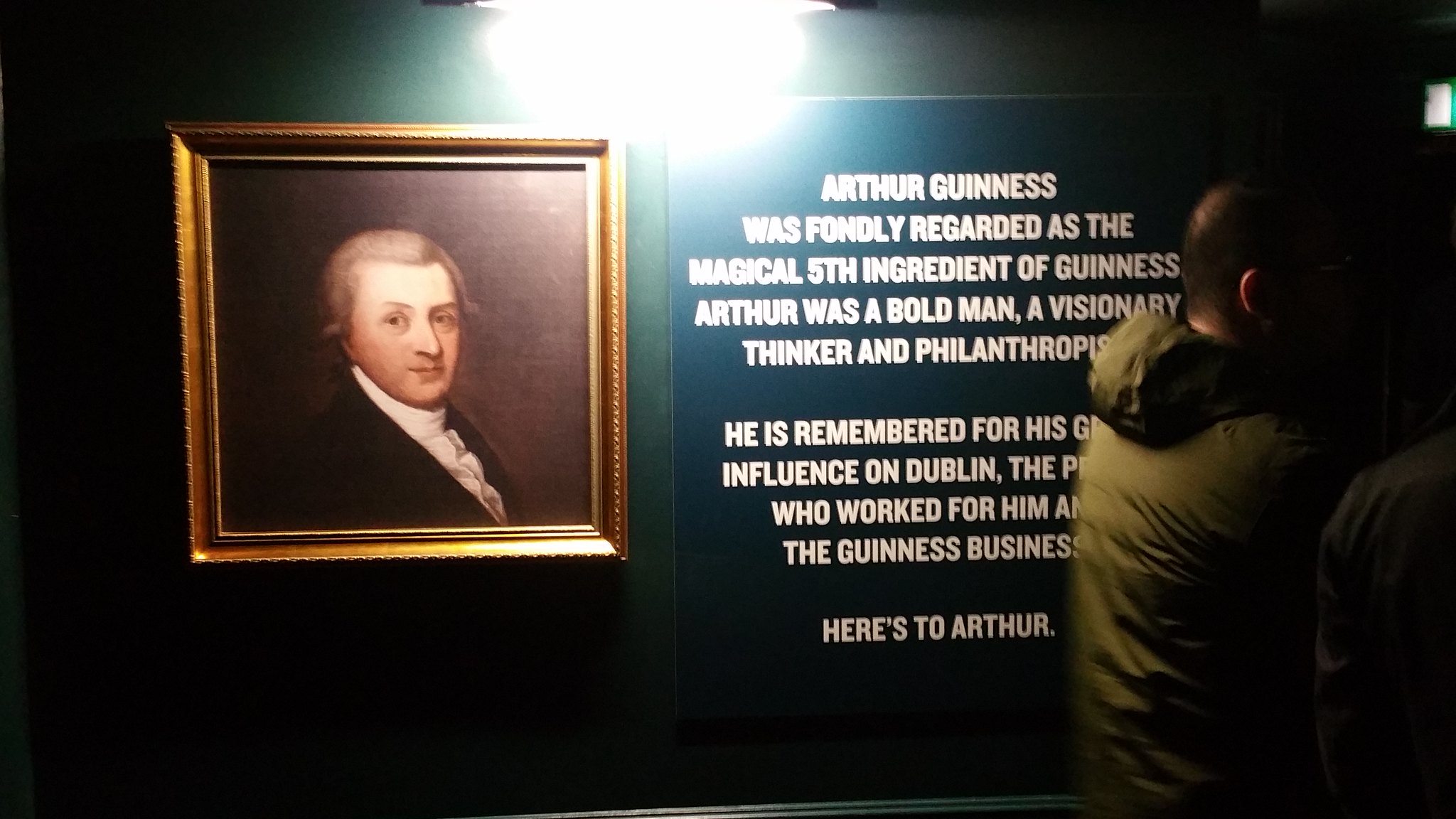In a dimly lit museum setting, a grainy photograph captures a historical exhibit. Dominating the museum wall on the left is a gold-framed portrait of Arthur Guinness, depicting him in colonial attire with gray hair, a white frilly shirt, and a black suit jacket. Adjacent to the portrait is a blue informational sign with white sans-serif text, partially obscured by the green coat of an onlooker whose face is shrouded in darkness due to the poor lighting. The sign praises Arthur Guinness as "the magical fifth ingredient of Guinness," highlighting his attributes as a bold visionary thinker and philanthropist. Despite the text being cut off, it alludes to his significant influence on Dublin and the people who worked for him at the Guinness business. A bright light at the top of the image adds to the overall poorly lit ambiance.